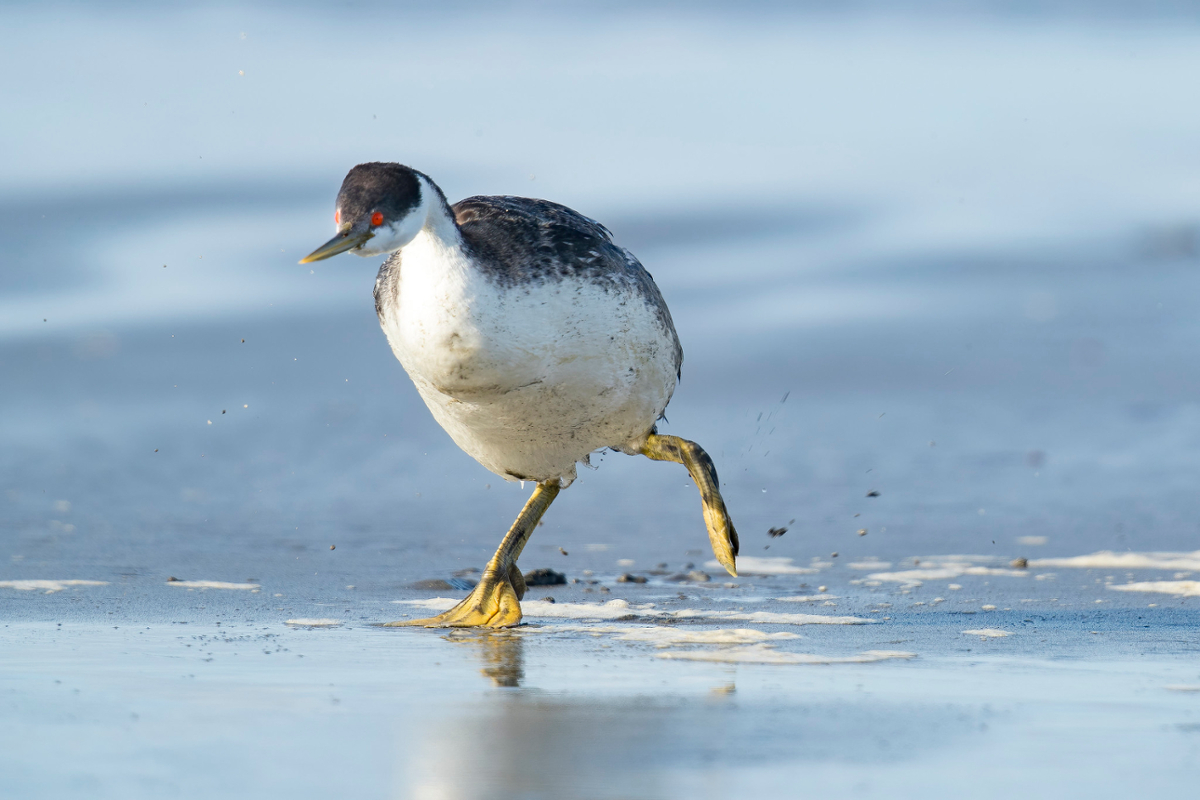The image features a young penguin-like bird as the focal point, walking along a seemingly icy shoreline. The bird has a striking appearance with its dark gray (black in some descriptions) head and back, a white underbelly, and bright red eyes. Its beak juts out, and it prominently displays yellow webbed feet—one of which is forward on the ice, while the other is raised, kicking up small patches of light blue ice and white patches as it moves. The surroundings feature a bluish-gray, unfocused background, suggesting either icy terrain or possibly a lakefront with pebbles and foam near the water's edge. The image captures the bird mid-stride, emphasizing its motion and the dynamic environment it inhabits.